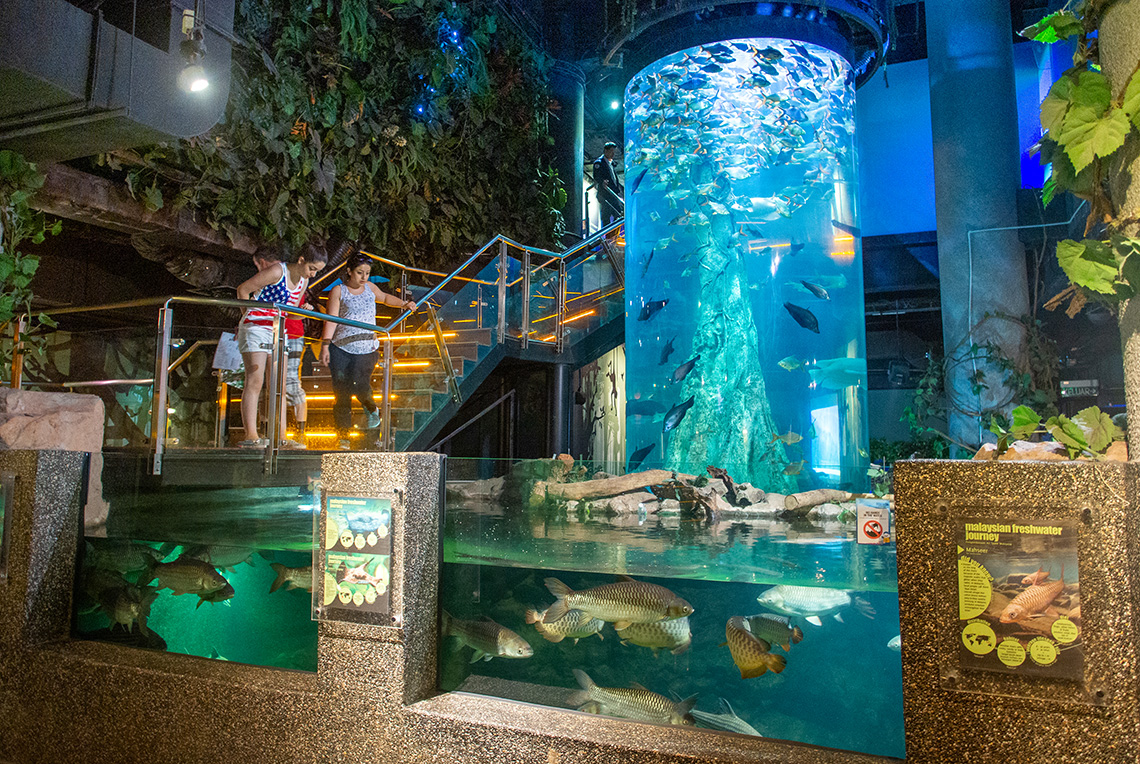The photograph showcases an elaborate and unique aquarium exhibit. In the forefront, a low glass wall is embedded in a granite-like stone barrier, fronting a large pool of clear blue water teeming with large gray and yellow fish. Multiple brown logs are scattered across the surface of the pool. Rising from the center of this pool is a tall, cylindrical aquarium filled with fish swimming in a circular motion. To the left of the scene, a staircase with a sleek glass and metal railing ascends, with several people, including two children and an adult, visible on the stairs and near the water's edge, observing the aquatic life. The background features walls adorned with hanging vines and strategically placed lights that illuminate the aquarium, enhancing the vibrant colors of gray, white, blue, green, red, brown, and white in the scene. The overall setting suggests a meticulously designed attraction likely found in an aquarium or a zoo.